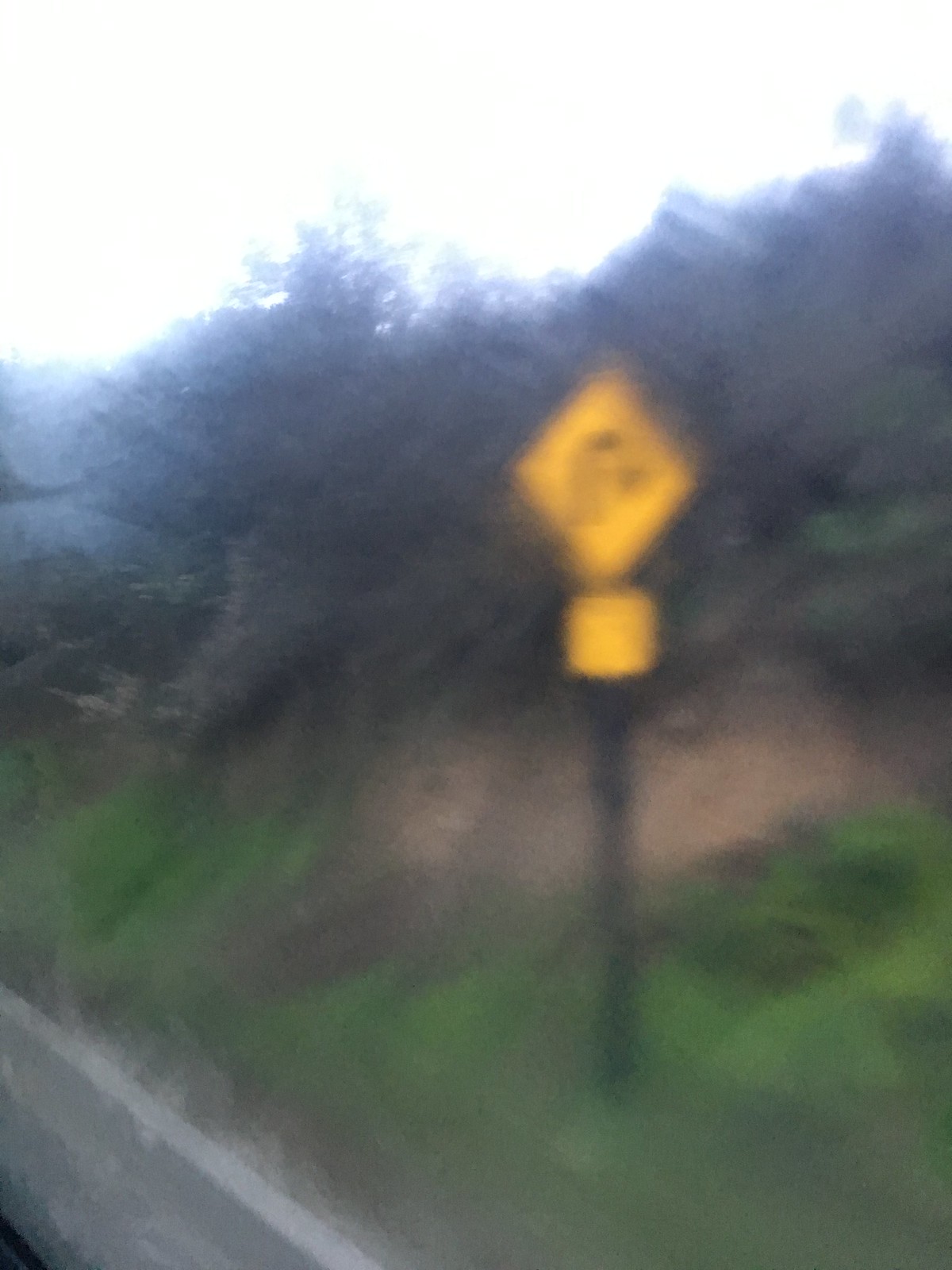This blurry, vertically oriented image appears to have been taken through the window of a moving vehicle, likely a bus or car, traveling along a highway or rural road. The camera's perspective shows the roadside scenery, which includes bushes, dense foliage, and grassy terrain. The sky above is completely overexposed, rendering it a bright, indistinct expanse. Central to the image is a black signpost that features two signs: a small yellow sign at the bottom and a larger, diamond-shaped sign above. Despite the blur, the diamond-shaped sign is discernible enough to reveal a U-turn symbol: an arrow pointing upwards before curving downwards to the right, indicating a U-turn ahead.